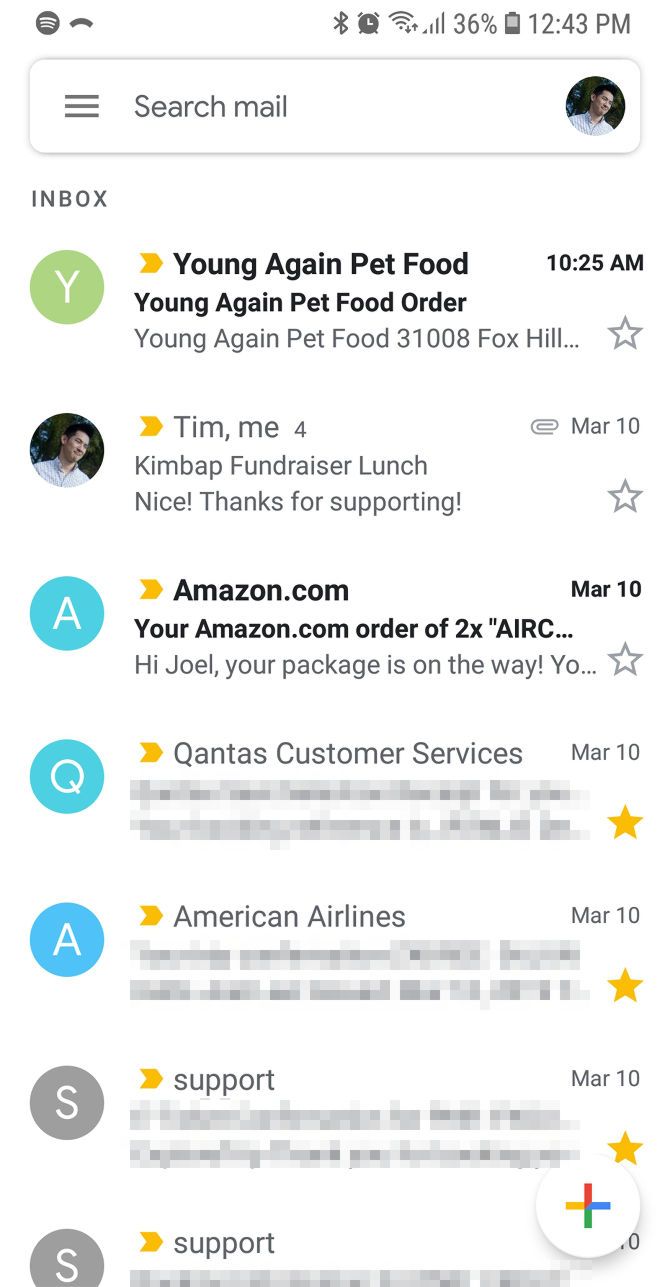The image depicts a specific section of an email webpage, focusing on the search mail area and a portion of the inbox. At the very top, the interface features a white rectangle with three horizontal lines on the left side, labeled "search mail" in gray letters. On the right side of this top bar, there's a profile picture of the webpage owner. Above this bar, system status indicators display the current time (12:43 PM), battery power at 36%, signal strength bars, and a Bluetooth icon.

Directly below the search mail bar, the inbox header is labeled "Inbox" in gray letters. The first visible message features a green circle with a 'Y', indicating the sender, "Young Again Pet Food," with the subject "Young Again Pet Food Order." 

Below this entry is a message from a person named Tim. The sender's photo is displayed, followed by "Tim, me," and the subject line reads "Kimbap Fundraiser Lunch," with the email content starting with "Nice. Thanks for supporting!"

Following Tim's message, there's another email from Amazon.com. It features a blue circle with 'YA' and the subject "Your Amazon.com Order of 2C ARC," with the message preview starting "Hi, Joe, your package is on the way."

Further down, there are additional messages from Qantas Customer Service, American Airlines, and two emails from support, though the specific contents of these messages are blurred and not readable.